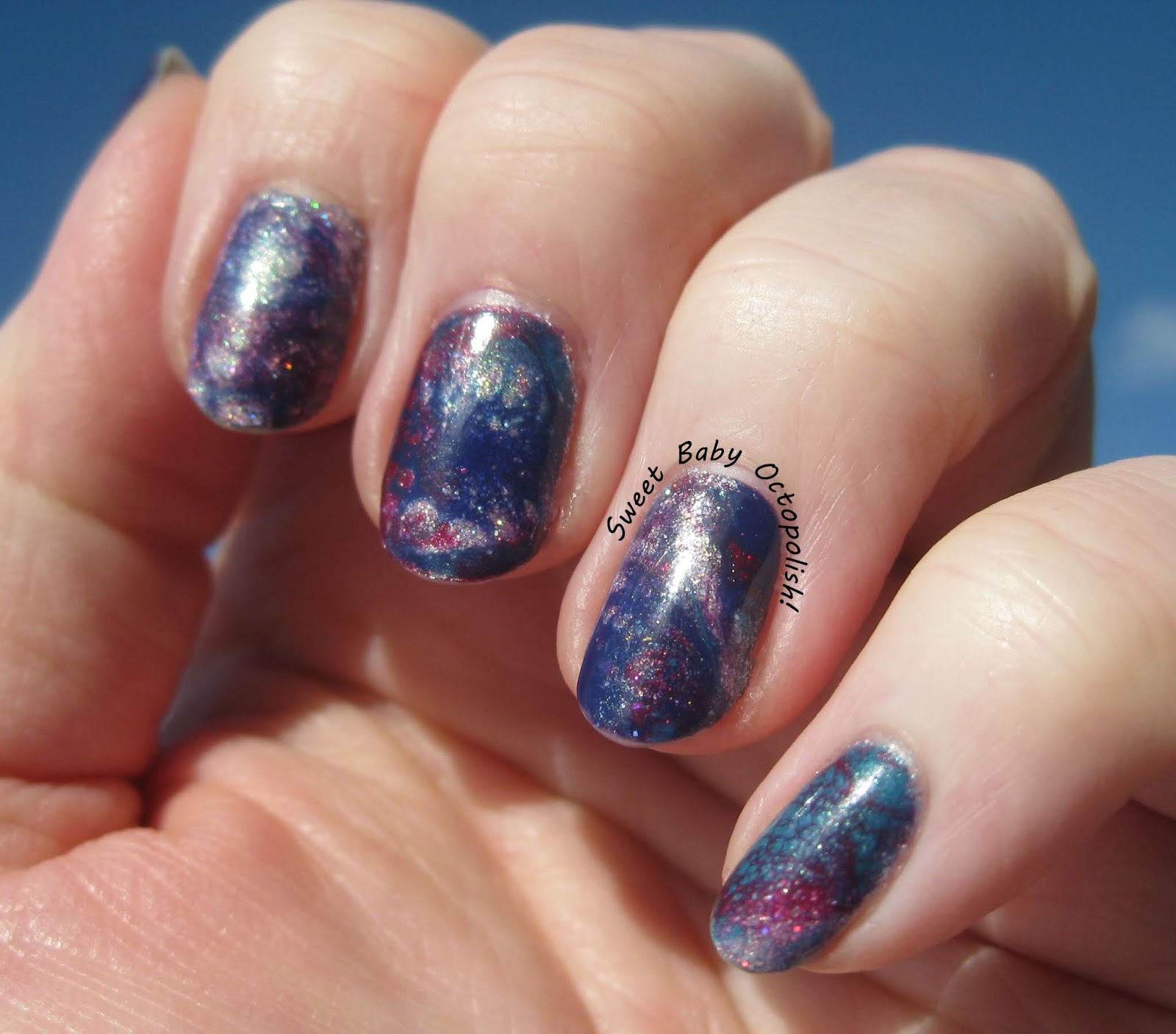A detailed photograph captures a white hand, likely a woman's, positioned against a bluish background. The hand is partially clenched, highlighting the four fingernails. The nails feature an intricate and eye-catching design: predominantly blue with silver metallic sparkles forming circles, and transitioning to a reddish base near the cuticle with additional metallic accents. Notably, above the nail of the third finger from the pinky, text reads "Sweet Baby Octopolish," suggesting a possible boutique nail salon's creative work. The combination of colors on the nails, including hints of purple, red, and pink with the sparkly elements, gives an impression reminiscent of a cosmic or space-themed manicure.